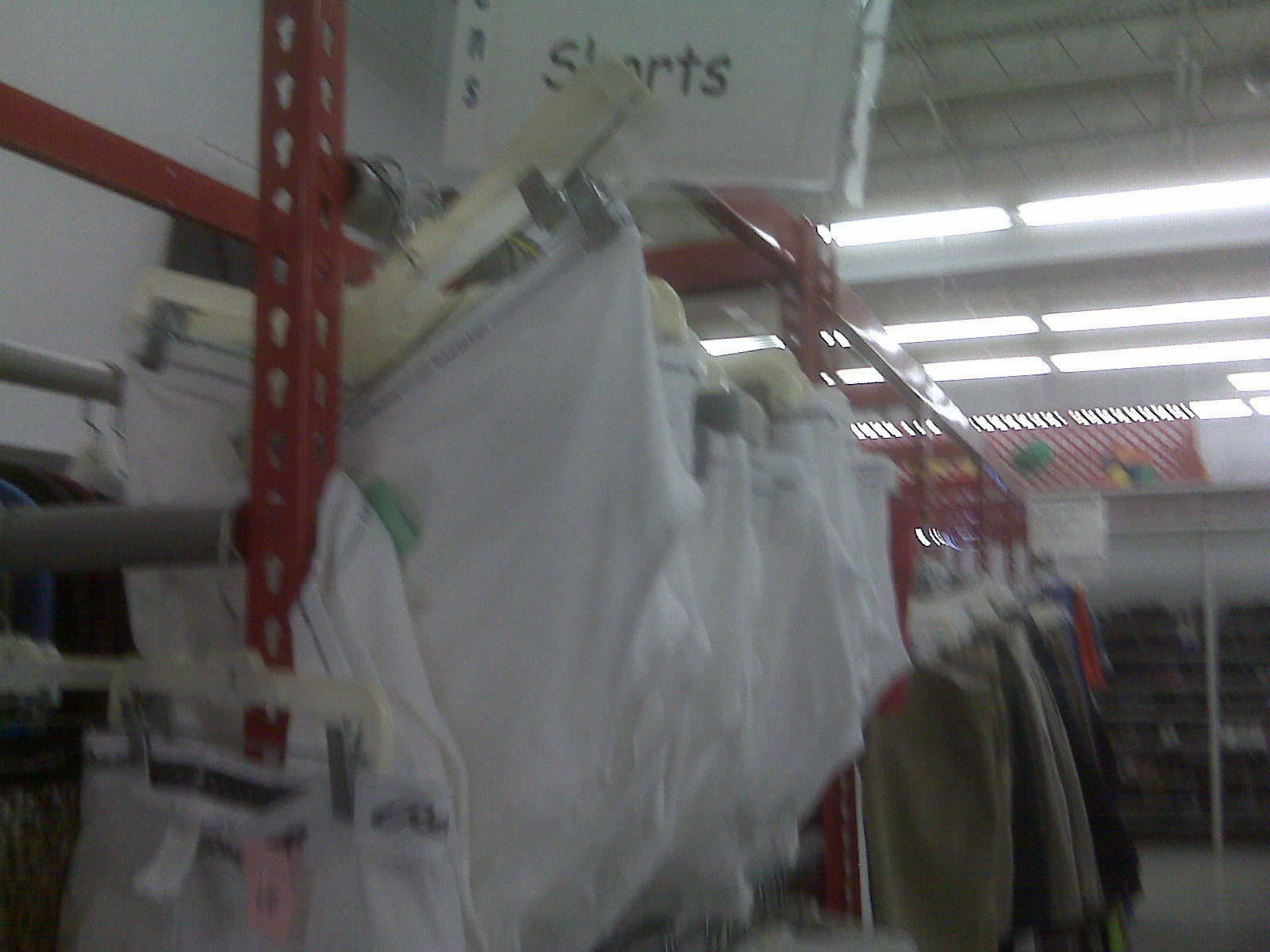The image depicts a section of a discount clothing store, focusing on an orange rack with multiple silver bars holding various hangers. Each hanger is clipped with white male underwear, which interestingly contradicts the laminated paper sign above that reads "SHORTS" in black text. The store is brightly lit by several rows of rectangular fluorescent lights attached to a white, metal ceiling adorned with white-painted scaffolding and support beams. The scene gives a utilitarian, industrial feel to the shopping environment.